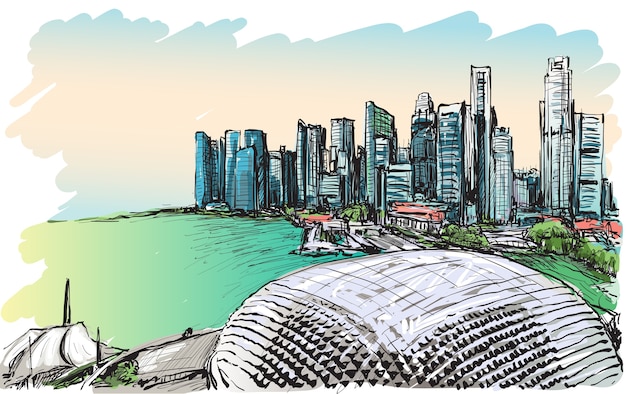This animated cityscape, rendered in a cartoonish style, features an array of tall skyscrapers clustered closely together, each adorned with numerous windows. The skyline showcases a variety of architectural designs, with a group of striking blue glass buildings forming a circular pattern at the top center of the image. Flanking these are a mix of tall white buildings with distinct black scribbles and a notable dark gray skyscraper.

In the foreground, a bustling harbor extends from the left side of the image, curving around in front of a charming neighborhood of smaller, red-roofed houses. The waterfront is characterized by muted tones of blue, green, and yellow, culminating in a vibrant mix that adds depth and texture to the scene. Near the very front, a prominent silver-domed sports stadium with a textured, triangular shape captures attention. Additionally, a large rock centered in the foreground and a few smaller rocks with leafy accents to the left provide a natural contrast to the urban environment. The sky is painted in soft watercolor hues of blue and rose, completing the picturesque, yet dynamic, cityscape.